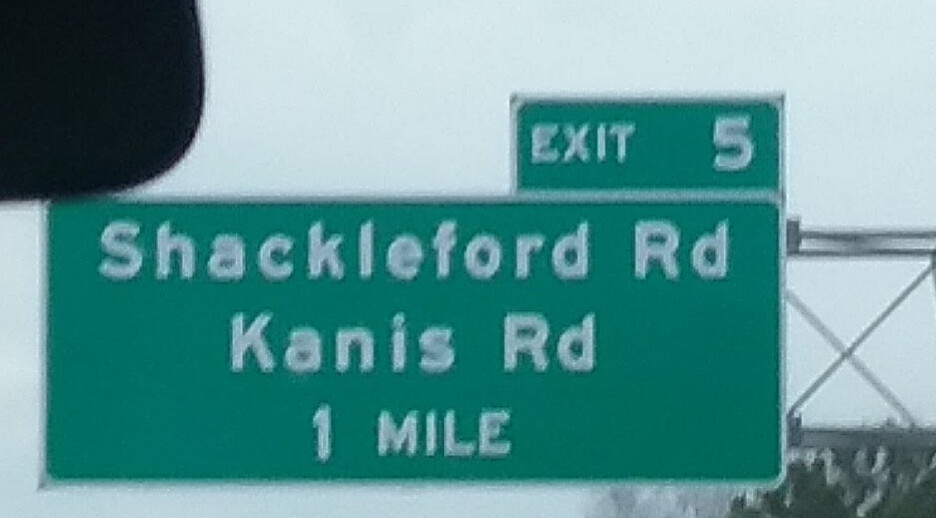The image captures a close-up view from inside a car, likely taken from the passenger seat, showcasing a detailed portion of the interior and a highway road sign. In the upper left corner, part of the car's rearview mirror is visible against a black background, suggesting this is near the front of the car, at the intersection of the driver's seat and passenger seat, up towards the ceiling. The main focus of the image is the highway sign, which is prominently positioned in the center. The sign is green with white borders and consists of two stacked rectangles. The smaller rectangle on top reads "EXIT 5" in capital letters. Below, the larger rectangle contains the text "Shackleford Road; Kanis Road" followed by "1 MILE," also in capital letters. Supporting the sign are grey metal horizontal bars, clearly visible on the left side of the image. Additionally, in the bottom right corner, there is a glimpse of a tree against a backdrop of clear blue sky that spans the top and bottom left of the image.